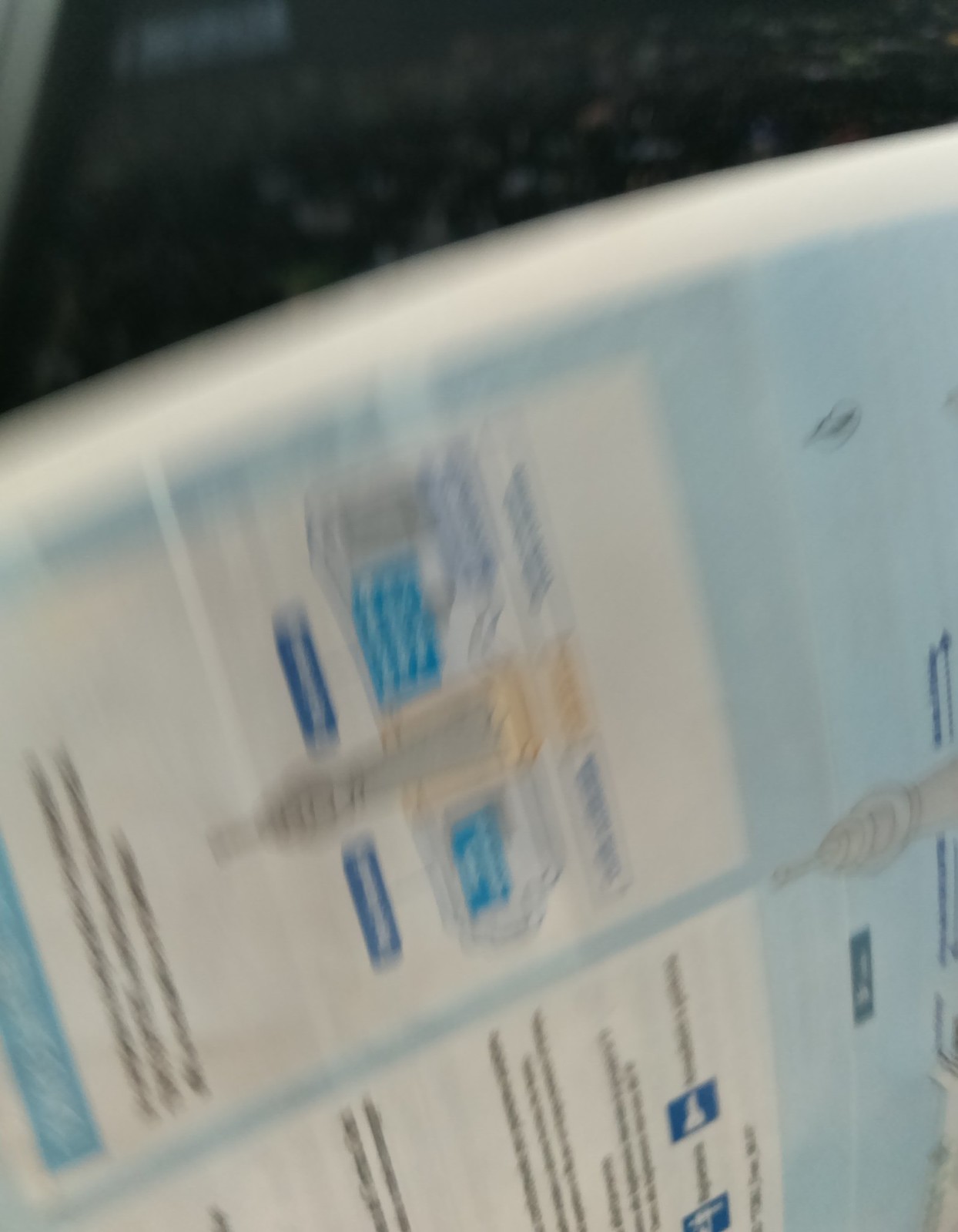This vertical, slightly blurry, close-up color photo appears to be an image of some sort of instructional artwork or guide. The image, captured sideways, features a blue background with several white boxes and includes an illustration that seems to depict a cross-section of a certain object. It’s unclear whether this object is a device, a food product, or something else due to the photo's blur and orientation. Text is present, but it is indistinguishable, making it difficult to ascertain the exact nature of the instructions.